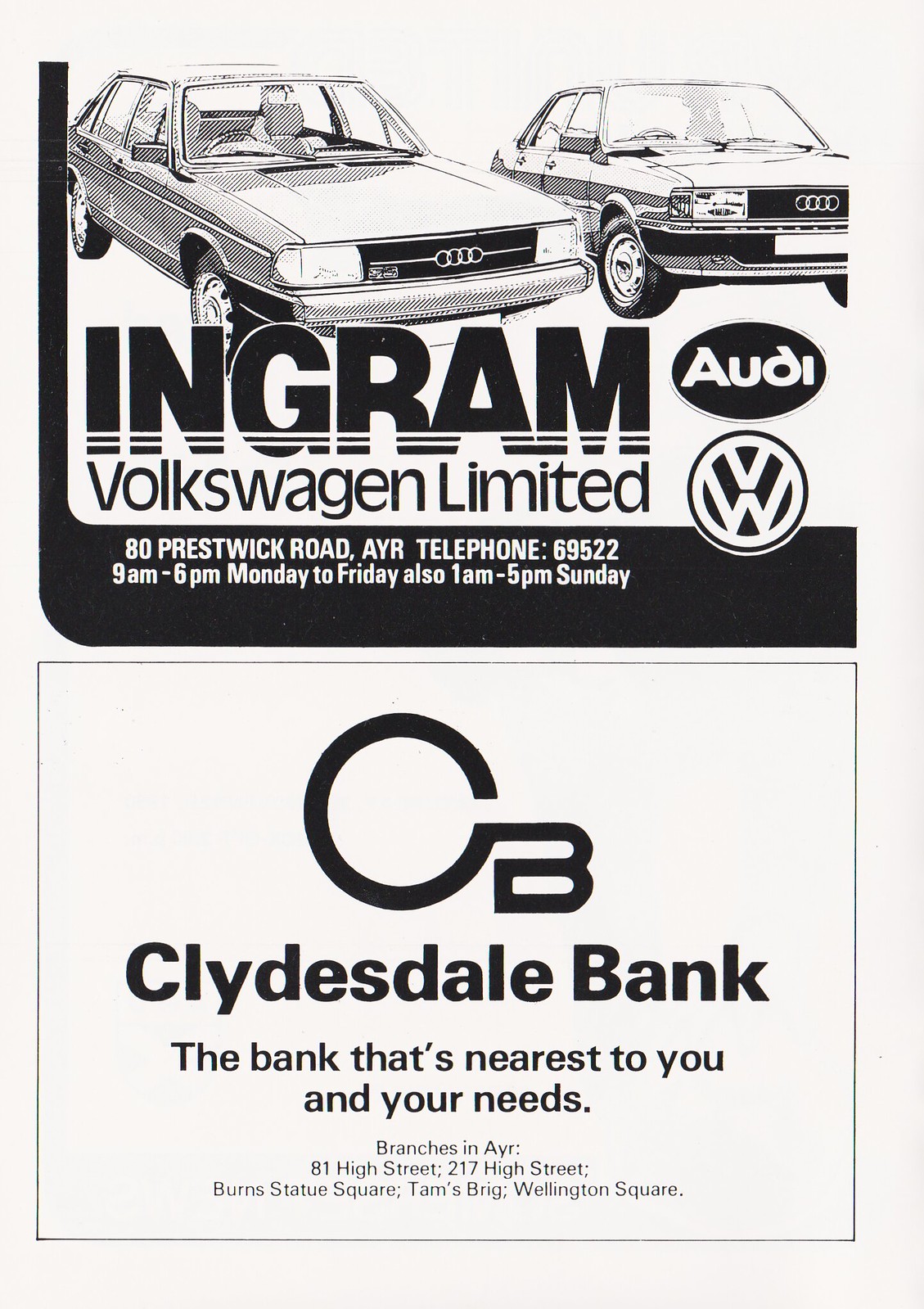This rectangular, vintage print advertisement, seemingly from the 1980s, appears to be a page from an old newspaper or magazine. The page is aged with a slightly brown tint around the edges. The ad is split into two main sections. The top section features illustrations of two older Audi sedans drawn in an ink style, giving them a distinctly 80s look. Above them, there is bold, black text that reads "Ingram Volkswagen Limited." To the right of this text, within a black oval, is the Audi logo, and adjacent to it in a white circle is the VW (Volkswagen) logo.

Below this, a black footer contains the dealership’s address and contact information: "80 Prestwick Road, AYR, telephone 695229, open 9 a.m. to 6 p.m. Monday to Friday, also 1 a.m. to 5 p.m. on Sunday."

The bottom half of the advertisement features another square, outlined in black, with a logo consisting of a large circular "C" connected to a capital "B," identifying it as Clydesdale Bank. Beneath the logo, the slogan "the bank that's nearest to you and your needs" is printed, followed by a list of branches: "Branches in AYR - 81 High Street, 217 High Street, Burns Statue Square, Tams Brigg, and Wellington Square." The overall design and content suggest this ad is both promoting the dealership and providing bank information, highlighting their local presence and services.